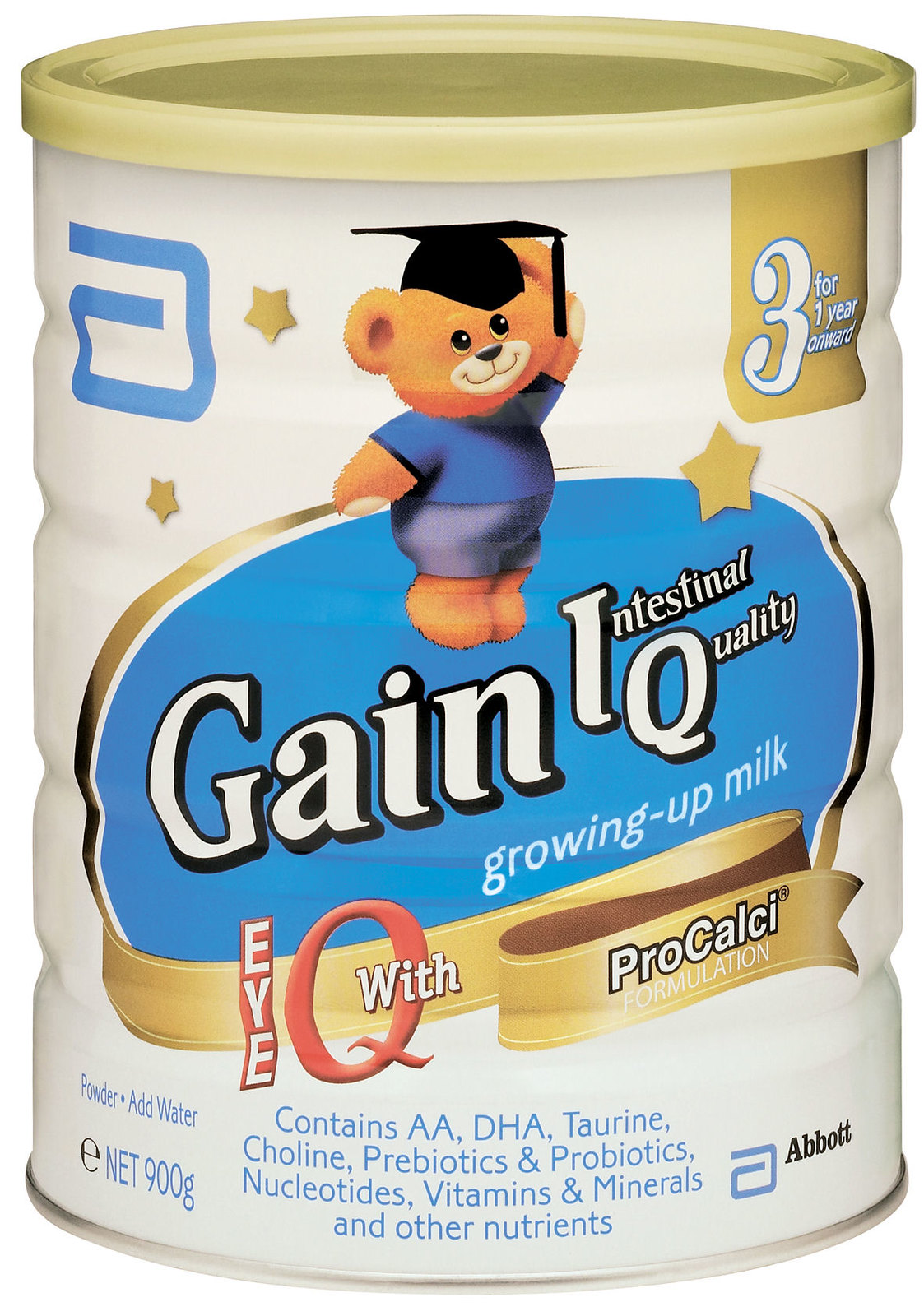The photograph showcases a container of baby formula. The container features a very pale yellow lid. Prominently, at the upper part of the container, there's a blue symbol visible. The main body of the container is adorned with white labels. 

A teddy bear character is part of the design, adding a friendly and welcoming touch. This teddy bear is depicted wearing a black graduation cap, symbolizing intelligence and learning. He is dressed in a blue short-sleeve shirt and matching blue shorts. 

The product name, "Gain IQ," is displayed prominently in white font against a blue background. Just below this, in a combination of red and white font, the label reads "IQ with Pro Calci formulation." The "Pro Calci formulation" text is designed in white font against a gold ribbon motif, adding an element of sophistication to the design. 

At the bottom of the label, in blue font, the text details the product's contents: "Contains AA DHA, Taurine, Choline, Prebiotics, Probiotics, Nucleotides, Vitamins and Minerals, and other nutrients." This list highlights the comprehensive nutritional profile of the formula, intended to support growing children.